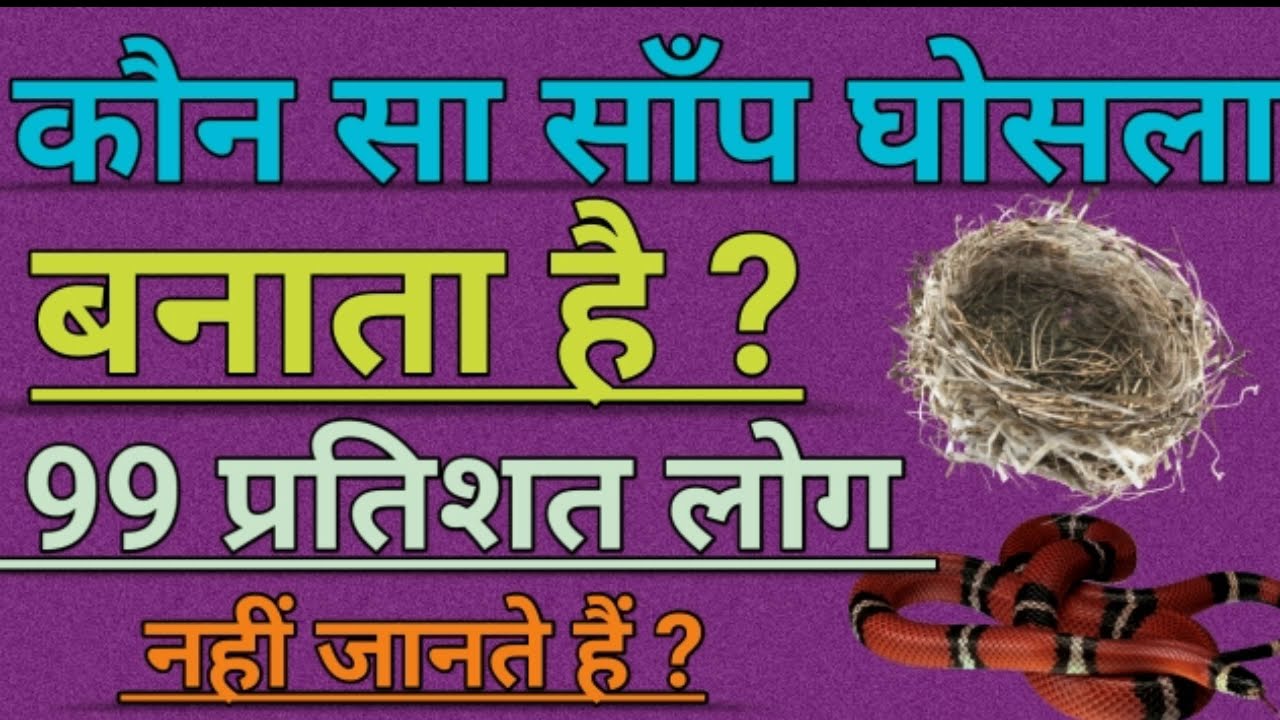The image appears to be an advertisement, possibly from a Southwest Asian or Middle Eastern region, featuring writing in a script that is unfamiliar. The text is bold and large, with four distinct lines of varying colors: the top line is blue with five symbols, the second line is yellow with three symbols ending in a question mark, the third line is white with the number 99 followed by two or three additional symbols, and the bottom line is orange. The background is a deep, solid purple. On the right side of the image, a bird's nest is depicted towards the center, while in the bottom right corner, a coral snake with striking red, black, and white bands is coiled, its head directed to the lower corner and its body winding upwards. The elements seem to be arranged somewhat randomly across the purple backdrop.